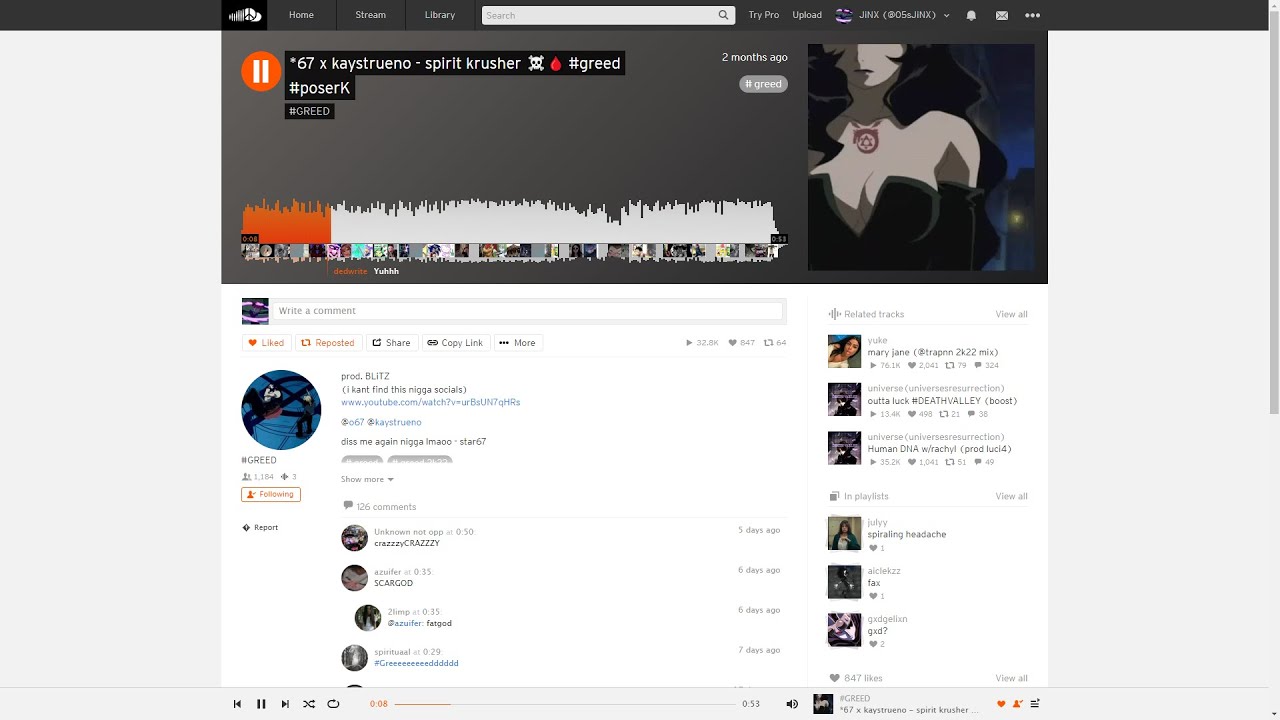In this image, we are presented with a zoomed-out view of a SoundCloud screen. Due to the zoom level, the text is not legible. At the top of the image, there’s a black background with the SoundCloud logo on the far left, followed by three categories, a search bar, additional categories, and a couple of white icons.

The track being played is "Spirit Crusher" by the artist KAYSTRUENO, with "Crusher" spelled with a 'K'. It is tagged with hashtags "#greed" and "#poser" (using a capital 'K' for "Kposer"). To the left of the track information is an orange circle with a pause icon, indicating the track is paused.

Below this, there is a waveform display that SoundCloud uses to visualize the music. The progress through the track is shown by a section of the waveform highlighted in orange, while the rest is in light gray. The track was posted two months ago, and the general background at this level is gray.

On the right side of the screen, there is an anime character of a woman with black hair. The entire bottom section of the image has a white background filled with numerous comments and suggested tracks. Both the left and right sides of the image feature a light gray background from top to bottom.